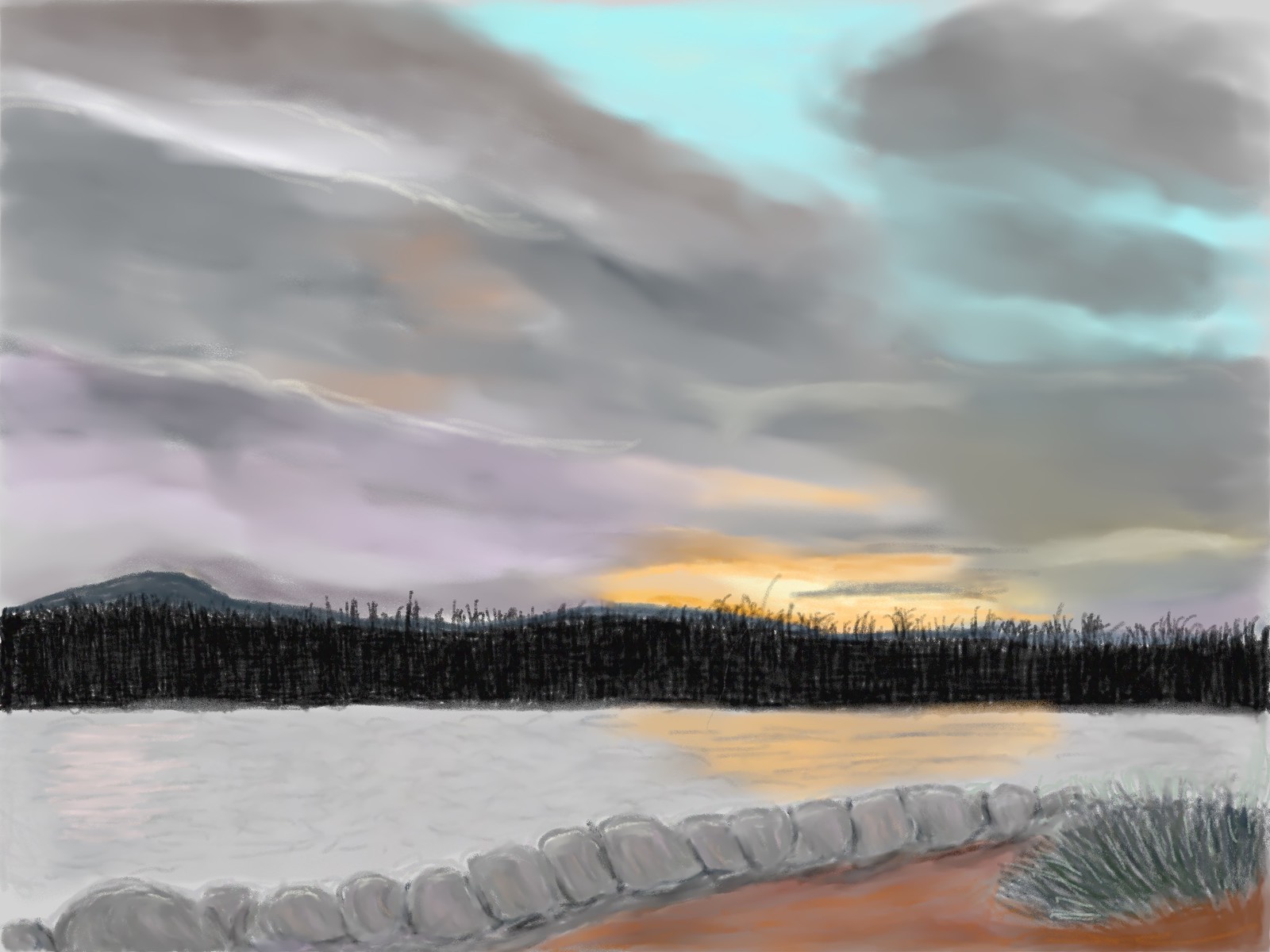The drawing depicts a picturesque skyline with a simple yet evocative color palette of grey, yellow, blue, brown, and green. In the bottom right corner, there's a small patch of brown ground adorned with a green bush. Above this, a grey stone embankment leads to the water, which is a pale blue, nearly grey, hue. The water features a yellow reflection of the sun, adding a touch of warmth to the scene. A dark, almost black, green strip suggests either a tree line or reed bed. Above this strip, the sky transitions from dark grey clouds downwards to a soft blue, with a small area where yellow sunlight breaks through, adding a hint of brightness to the otherwise muted skyline.